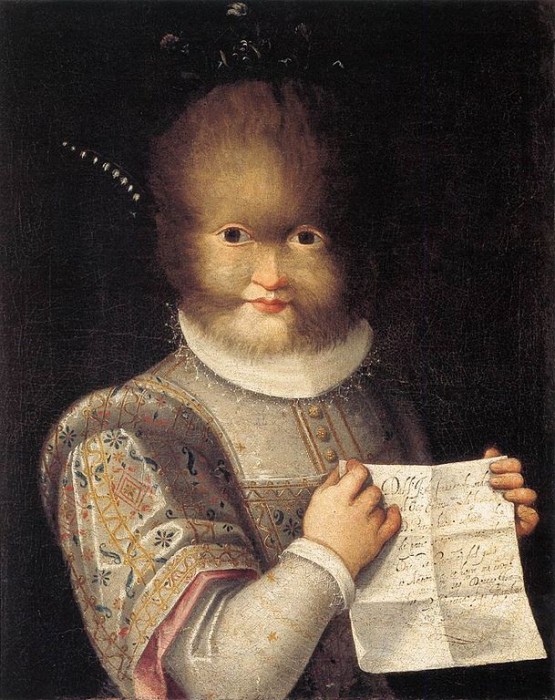The image depicts a highly detailed, vintage-inspired painting of a person whose face is directed towards the viewer while their body is turned to the right. The individual is holding up a white piece of paper, prominently displaying it. They are dressed in an antique-style, short-sleeved gown layered over a white shirt. The person, seemingly a woman, has her face partially obscured by voluminous hair. She is adorned with a striking, black, crown-like headpiece characterized by sharp, peaked elements. The overall aesthetic suggests an artwork steeped in historical and fantastical elements.